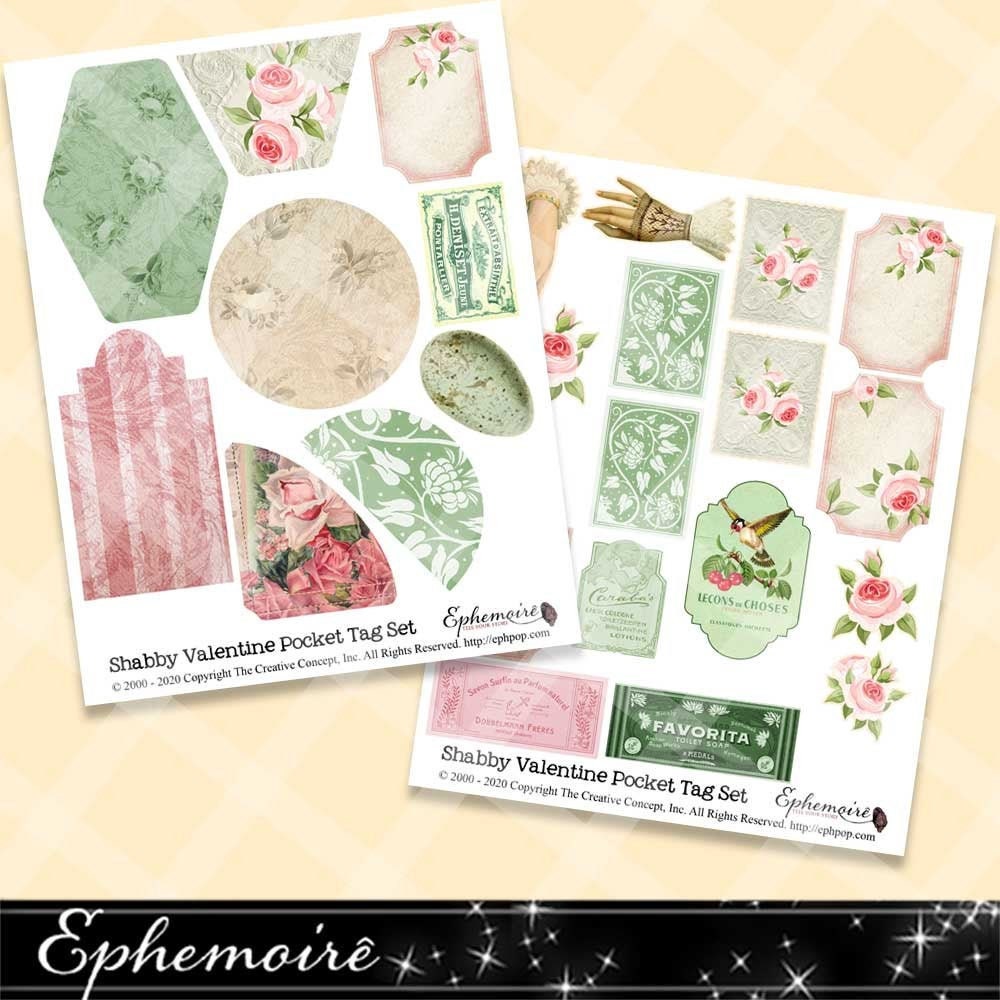This image features a shabby-chic Valentine pocket tag set. The background is a light tan color with a subtle diamond pattern. At the bottom of the image, a black banner with white stars and cursive text reads "Ithamori Moray." Above the banner, on both the left and right sides of the image, are two overlapping sheets of Valentine tags. These sheets are adorned with intricate floral designs, predominantly in pinks and greens, with patterns of roses, hummingbirds, and hands with black markings. 

The top-left sheet contains a variety of tag shapes, including rectangular, circular, and fan-shaped tags, featuring green flowers, pink roses, and a green oval. The top-left sheet slightly overlaps the bottom-right sheet, which also showcases floral patterns and an image of a hummingbird, with a similar color palette. Each sheet has around nine to several tags, indicating variations in their sizes and designs. 

At the bottom of the sheets, it’s noted “Shabby Valentine Pocket Tag Set Ithamori 2000 to 2020,” accompanied by copyright information from "The Creative Concept Ink, All Rights Reserved," along with a website. The image overall gives a vintage, romantic, and detailed feel, emphasizing the artistic and elaborate nature of the tags.